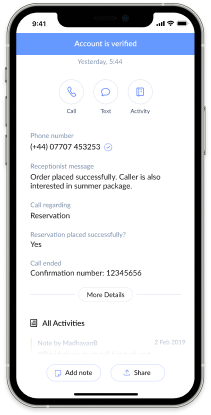This image shows a smartphone screen displaying detailed information on a recent communication. At the top, the screen displays the current time along with the Wi-Fi signal strength and battery life indicators. Below these indicators, there is a blue banner with white text that reads "Account Verified."

The main content of the screen includes a header stating "Yesterday, 5:44 PM." Following this, three buttons are displayed labeled "Call," "Text," and "Activity." The screen also shows a phone number: "+44-077-07-453-253," accompanied by a blue checkmark indicating verification.

The content reveals details of a receptionist's message stating that an order was placed successfully. It also mentions that the caller expressed interest in a summer package. Further down, there is a note about a call related to a reservation, which was successfully placed, along with a call ending confirmation number: "12345656."

A black "More Details" button is present, along with text displaying "All Activities." Below this, there is additional information, including the date "2nd of February 2019."

At the bottom of the screen, two buttons are present: one is labeled "Add Note," featuring a blue note icon and black text, and the other is a share button with an upward-pointing arrow and a blue underline. The background of the screen is predominately white, with black text and various functional buttons.